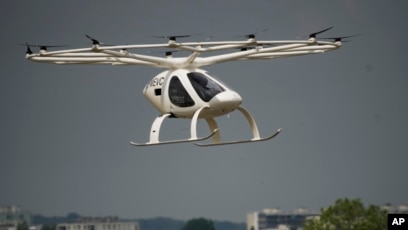In this photograph, a white drone-like aerial vehicle, which resembles a small helicopter, is seen hovering against a gray sky, about 10 to 20 feet above the ground. The vehicle is equipped with numerous small rotors connected to a circular structure at the top, featuring at least a dozen blades and possibly driven by electric motors. Its body is oval-shaped with tinted black windows on three sides. The landing gear consists of four white legs with ski-like footing. Below the drone, at the bottom of the image, the tops of trees and buildings are partially visible. In the bottom right corner, there's a black box with white "AP" initials, likely referring to the Associated Press. This detailed scene suggests the drone is capturing or monitoring something, possibly for a news agency.